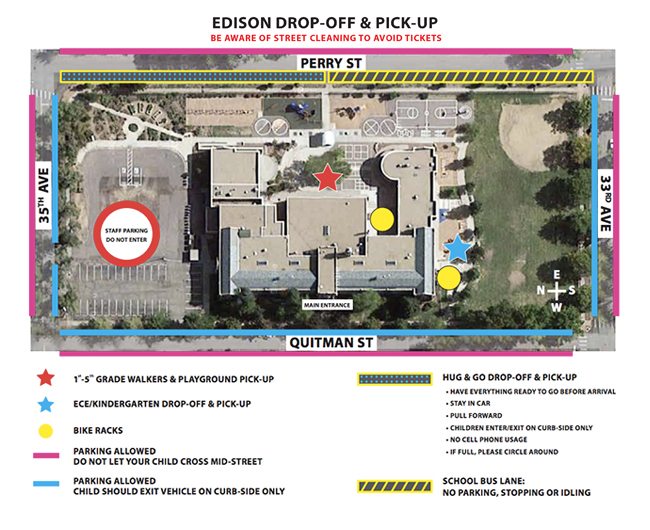The detailed map of Edison School showcases essential areas and guidelines for an organized drop-off and pickup system. Labeled clearly, the map marks out sections with distinct symbols and colors: red stars indicate the first- to fifth-grade walkers' drop-off and playground pickup zones, while a blue star marks the kindergarten (ECE) drop-off and pickup area. Yellow circles represent bike racks, scattered around the school premises. Parking instructions are indicated with various symbols: pink lines for general parking, blue lines for curbside-only parking areas, and no-parking zones around the school bus lane, which is highlighted with a yellow border and black middle, featuring blue dots.

The aerial view also provides street names to help orient parents: 35th Avenue on the left, Perry Street at the top, 33rd Avenue on the right, and Quitman Street at the bottom. Specific instructions are provided to avoid street cleaning tickets, ensure children only exit on the curbside, and maintain a smooth flow of traffic with the "Hug-and-Go" lanes. These lanes, bordered in yellow with black in the middle, require parents to stay in their cars and pull forward as spaces free up, with strict no-cell-phone usage policies. Additionally, the staff parking lot on the left side is marked as a "Do Not Enter" zone for parents.

Emphasizing safety, the map advises against allowing children to cross Mid Street and highlights the importance of preparedness before arrival to facilitate quick drop-offs. The overall layout includes expansive green, grassy areas and trees, typical of a suburban school, providing a clear, organized, and safe arrival and departure process for Edison School students.